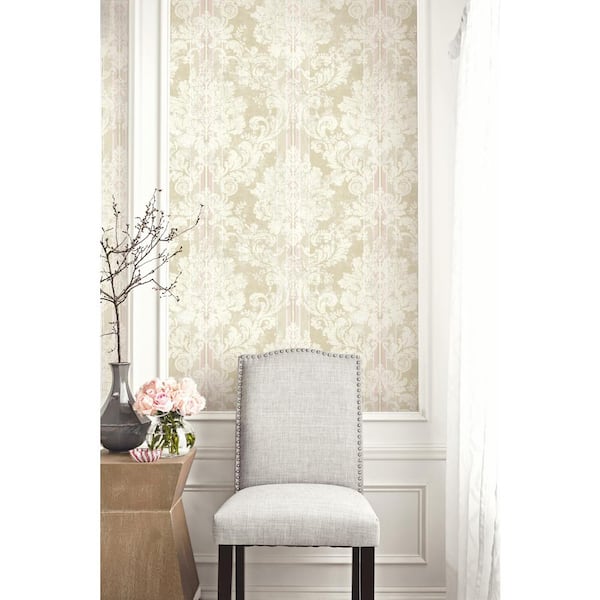The image depicts a sophisticated, cozy setting, possibly within a home or an office. It showcases a central gray chair with a cream-colored cushion and back, adorned with decorative nail studs, and perched on brown legs. The chair is prominently positioned against an intricate wall divided by wainscoting below and adorned with ivory and light brown floral wallpaper above. To the left of the chair stands a brown wooden side table. Atop the table rests a gray vase containing a flowering branch, a smaller clear vase filled with pink roses, and an ornamental glass dish with alternating pink and red stripes. On the right side of the scene, sheer white lace curtains partially obscure a window, allowing soft light to filter into the room. The color palette features elegant tones such as gray, brown, black, pink, green, cream, and ivory, contributing to the room's tranquil and stylish ambiance.